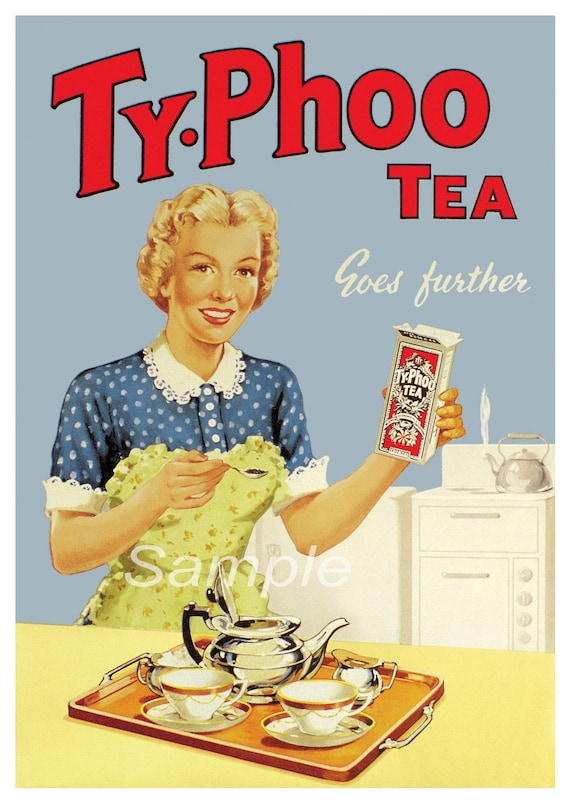This image is an advertisement reminiscent of the 1950s or 1960s, featuring a vertically aligned rectangular layout that resembles a poster or sign. At the top, bold red block letters outlined in black spell out "Typhoo Tea" with an intriguing typographic detail: T-Y followed by a dot and then P-H-O-O. Beneath this, in elegant white cursive, the slogan "goes further" is inscribed, emphasizing the product's promise.

The central figure is a cheerful woman with short, curly blonde hair, likely of Caucasian descent. She radiates a vibrant smile, clad in a blue shirt adorned with white polka dots, featuring white ruffled sleeves and a matching collar. Over her attire, she wears a green apron, possibly of a pale yellow or beige hue. In her left hand, she proudly displays a red and white box of Typhoo Tea, and in her right, she holds a spoon, presumably containing black tea.

Positioned in front of her is a yellow countertop, upon which rests a brown serving tray with silver handles. The tray holds a silver teapot, accompanied by a creamer and a sugar bowl, as well as two teacups waiting to be filled. The background features a blue wall with a white stove visible on the right-hand side, adding to the domestic ambiance of the scene. The word "sample" is printed in white across the center of the image, making this a striking and nostalgic advertisement for Typhoo Tea.